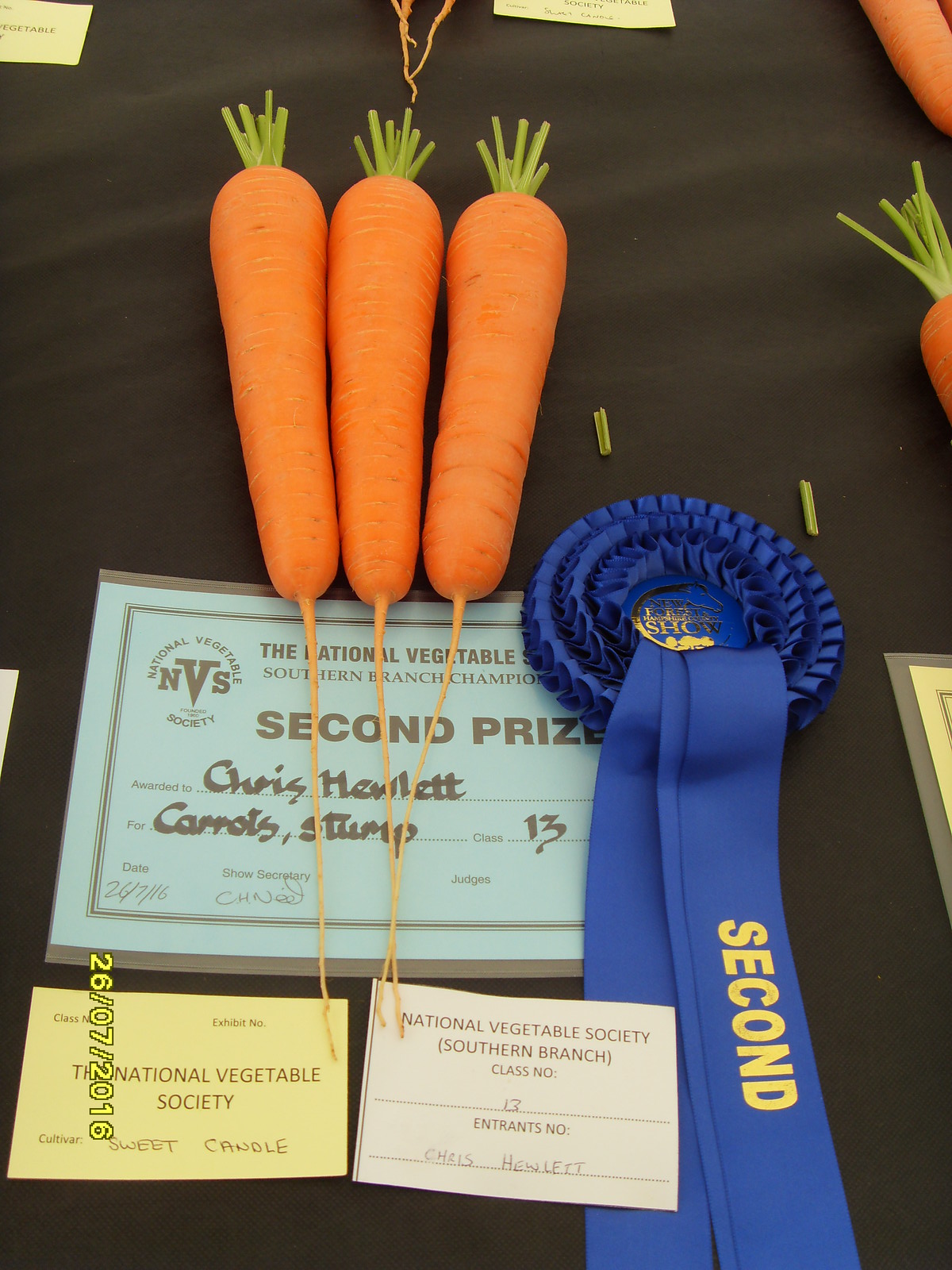This image captures Chris Hewlett's award-winning entry in the National Vegetable Society Southern Branch Championship, where his impressive carrots earned a well-deserved second prize. The photograph prominently features three robust and healthy-looking carrots with vibrant green stems and elongated, orange taproots, arranged neatly on a black tablecloth. Placed beside the carrots is a distinctive blue ribbon, with "SECOND" emblazoned in gold, symbolizing his achievement. Also visible is an official ticket and business cards from the National Vegetable Society, indicating his participation in Class 13. In the upper right corner, the tip of another carrot peeks out. The detailed setup underscores the quality of Chris Hewlett's produce, highlighting his success in growing prize-winning carrots.